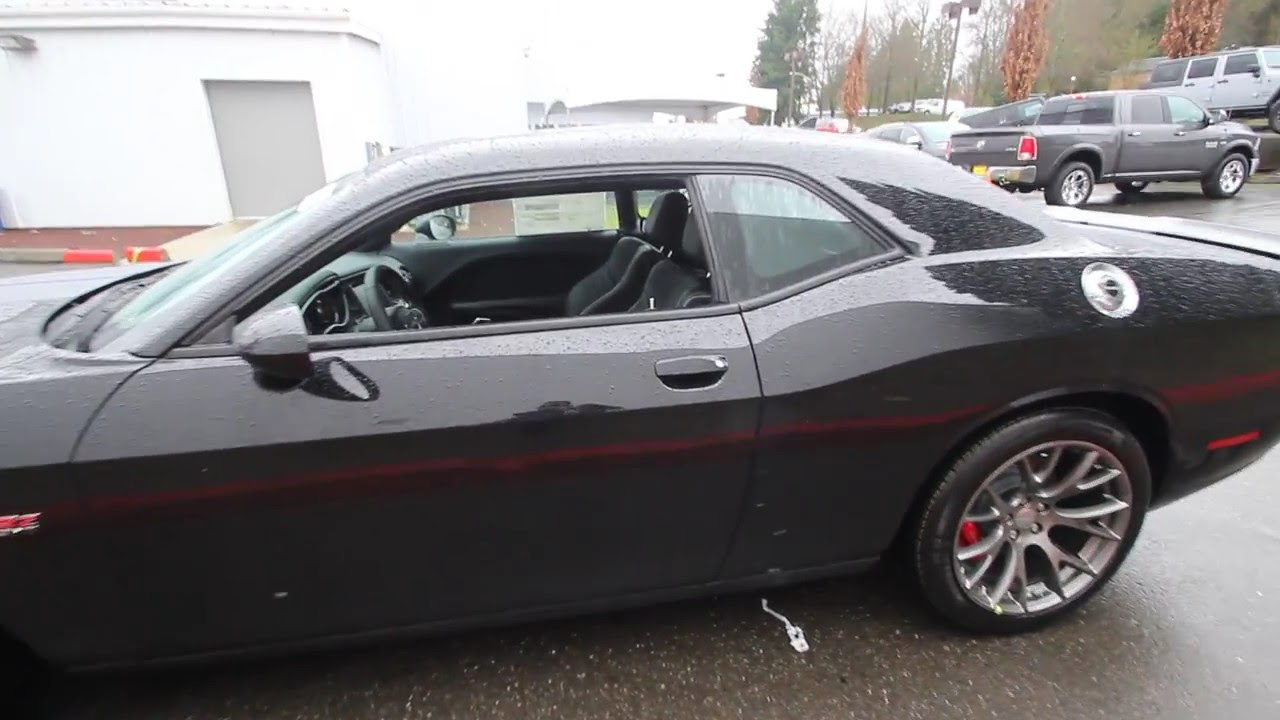The image captures a grey, rainy day in a parking lot with wet pavement and overcast skies. Foremost in the frame is a sleek black sports car adorned with silver rims and black tires, with red lettering visible on the front left side. The car's windows, both on the driver's side and passenger's side, are rolled down, revealing a black interior. Water droplets speckle the car's surface. Right next to the sports car stands a white building featuring a grey door and a square light. Further into the background, there is a grey pickup truck with black tires and silver rims, carrying a yellow license plate, and a grey and black Jeep parked slightly higher up. In the far distance, a white tent can be discerned. The right background shows a mixture of green and brown trees with thin trunks. Additionally, what appears to be an electrical cord extends a short distance from the car to the wet parking lot pavement.